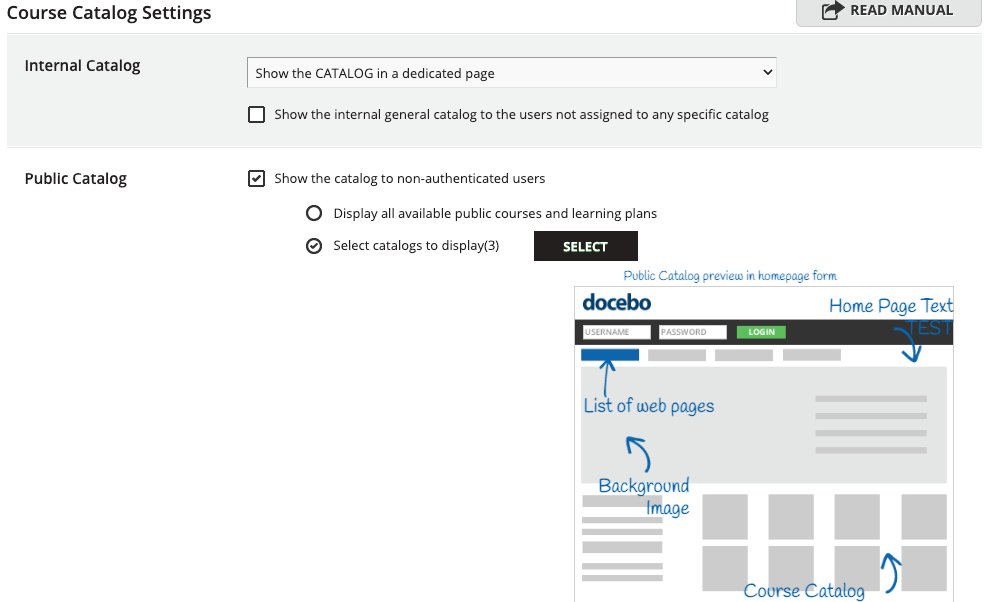This image showcases a detailed settings menu for a course catalog interface.

At the very top left, prominently displayed in bold letters, is the title "Course Catalog Settings." To the top right, there is an option labeled "Read Manual," accompanied by a PDF icon, which can be clicked to download a manual.

Below this, a long, light gray rectangular box displays the text "Internal Catalog," with an associated dropdown bar that offers the choice "Show the catalog on a dedicated page." Beneath this, there is a checkbox with the label "Show the internal general catalog to users not assigned to any specific catalog."

Further down, the section titled "Public Catalog" includes an option for "Show the catalog to non-authenticated users." This section also features a display for "Available public courses and learning plans." Adjacent to this, there is an option titled "Select catalogs to display," next to which is a black box with the word "Select."

In the center of the screen, there is a visual mockup or example layout, demonstrating how the eventual page will be organized. This mockup includes various elements, such as a blank box with several empty spaces and arrows providing guidance. At the top of this mockup, it is labeled "Home Page Text," with an arrow pointing to a section indicated as "List of Web Pages," consisting of four horizontal bars representing the web pages.

Another arrow indicates a "Background Image" placeholder, denoted by a blank box where a background image can be added. Additionally, there is a section for the "Course Catalog," highlighted by a series of eight gray boxes, indicating where the courses will be displayed on the final page.

Overall, the image offers a comprehensive view of how to configure various settings and layout options for a course catalog, guiding users through setting up internal and public catalogs, associating display options, and customizing the visual arrangement of the catalog page.